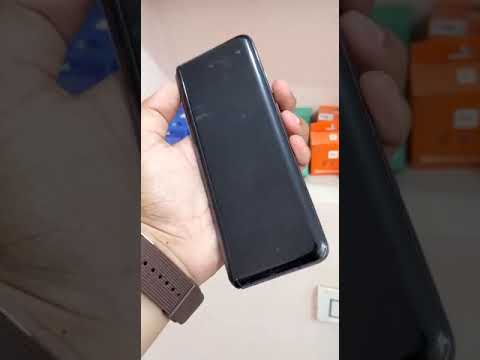The image features a detailed close-up of a white person's hand holding an upside-down black smartphone, centrally framed by two tinted zoom-in sections on either side. The hand, adorned with a brown watch on the wrist, has the thumb placed in the top left corner of the phone, with three fingers partially visible, showing the fingernails as they wrap around the device. The background reveals a light, flesh-colored wall. Behind the phone, to the left under the thumb, a blue object is discernible. To the right, near the fingers, there is a stack of orange boxes, with varying shades of orange and white labels on them. Additionally, a white square with a central button, framed by a gray square, is situated in the bottom right of the background. The side sections of the image, although grayed out, mimic the central photo, providing a zoomed-in view of the same scene.